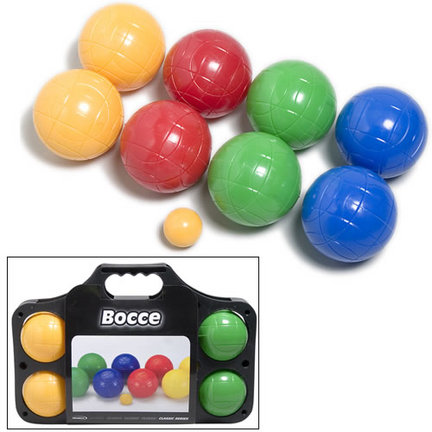The image is a detailed advertisement for a bocce ball set on a white background, featuring two parts. The top section showcases a close-up of the bocce ball set, consisting of eight shiny, textured balls—two yellow, two red, two green, and two blue—arranged diagonally, with a smaller yellow ball positioned between the red and green balls. The smaller ball, likely essential for the bocce game, resembles a larger marble in size. The balls appear to be made from a very hard, glossy plastic. Below this, inset on a black border, is an image of the same bocce ball set in its black carrying case. The case, bearing the word "bocce" in white text, features a handle at the top and an illustration of the included balls. In the visible sections of the case, the two yellow balls are seen on the left side, and the two green balls are on the right side. An indistinct text is present at the bottom of the carrying case.